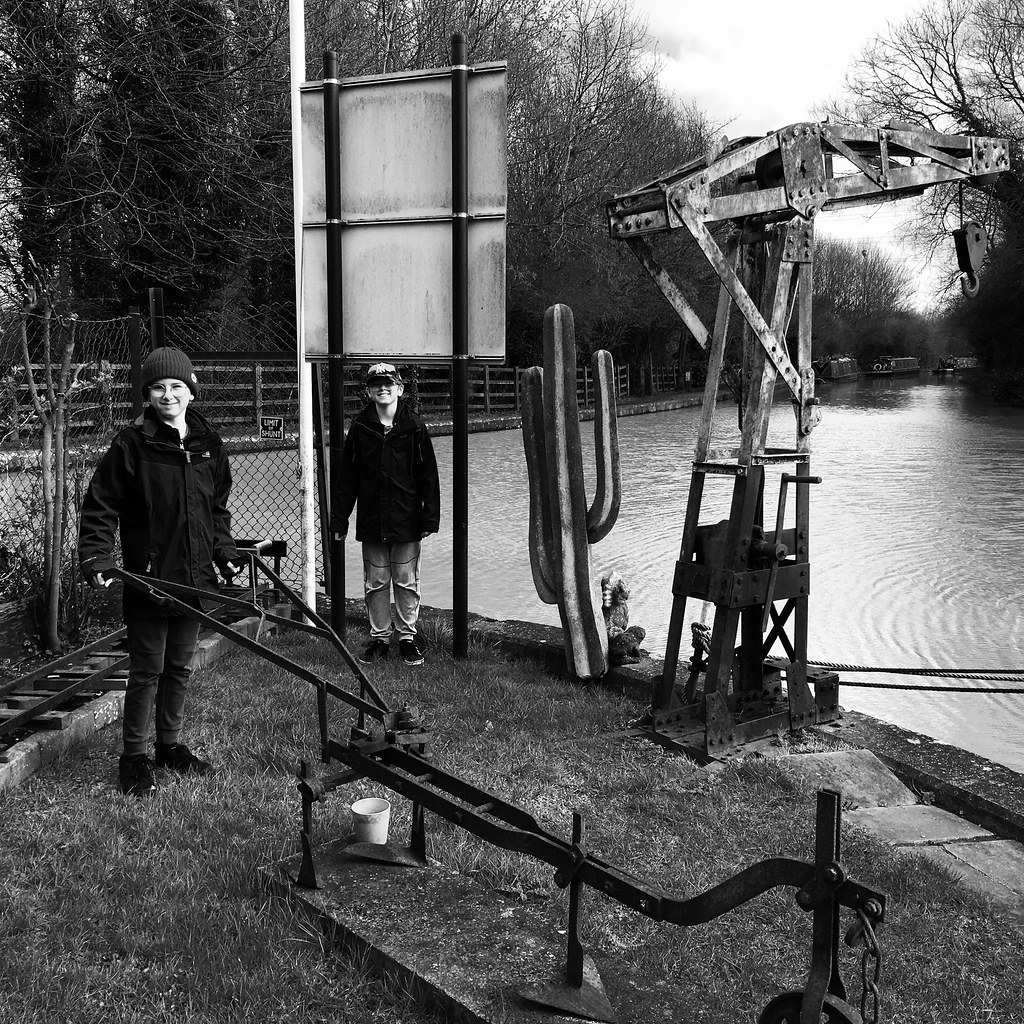The black-and-white photo captures a modern scene by an artificial canal, where two young boys stand prominently in the foreground. The boy on the left, wearing a beanie, holds a peculiar metal contraption featuring two handlebars, while the boy on the right, donned in a baseball cap, stands beside a reversed metal sign. Both are surrounded by an assortment of metal tools and structures, including a small riveted crane with a hook hanging over the water's edge. The canal stretches into the distance, lined with canal boats and bordered by a wooden fence on the left side, which transitions into a chain link fence near the boys. The wintery setting is evident from the leafless trees in the background, and the rippling water suggests a recent rainfall. Additional details include a light railway track on the left, and the intriguing presence of a cactus or garden structure near the crane.